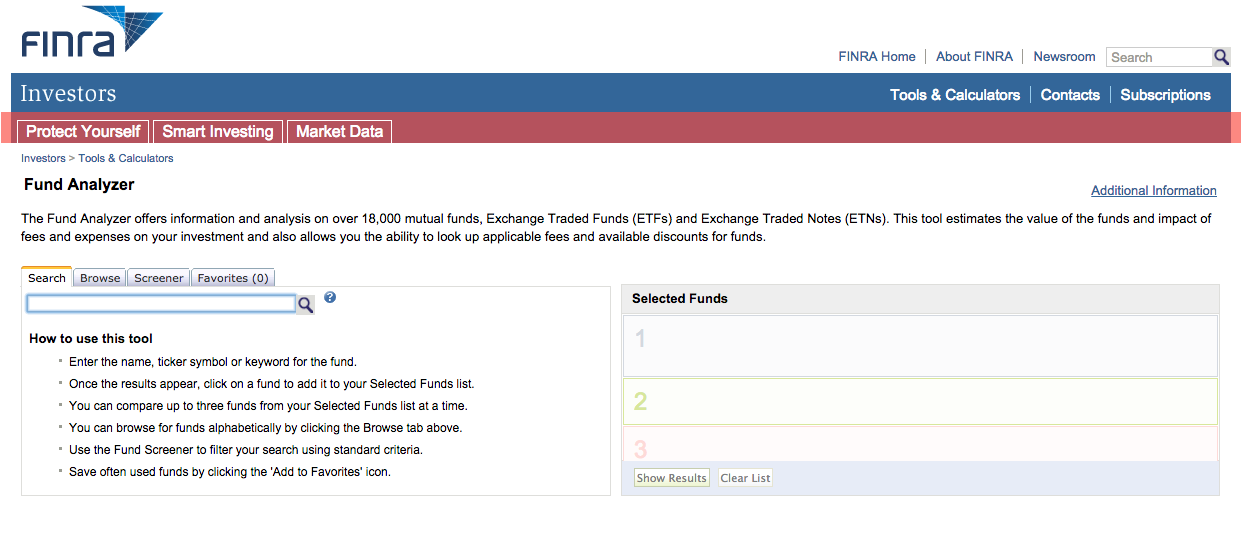A detailed description of the FINRA investor website image:

The webpage features a large, clean white square as its main background. At the top-left corner, “FINRA” is prominently displayed in blue lettering. On the top-right side, there are several navigation options including "FINRA Home," "About FINRA," "Newsroom," and a search function. Boldly placed at the top-left of the page is the section title "Investors."

On the right side, forming a second column towards the page top, there are quick links for “Tools and Calculators,” “Contacts,” and “Subscriptions.” Situated further down on the left side, in a burgundy box with white lettering, there are three key navigation options labeled "Protect Yourself," "Smart Investing," and "Market Data."

Dominating the central part of the page is the main feature – the Fund Analyzer. This tool offers extensive information and analysis on over 18,000 mutual funds, exchange-traded funds (ETFs), and exchange-traded notes (ETNs). It helps users estimate the value of these funds while evaluating the impact of fees and expenses on their investments. Additionally, the Fund Analyzer provides the functionality to look up applicable fees and discover available discounts for different funds.

At the bottom of the page, depicted in black lettering, are instructions on how to utilize the tool effectively, along with options to select specific funds for analysis.